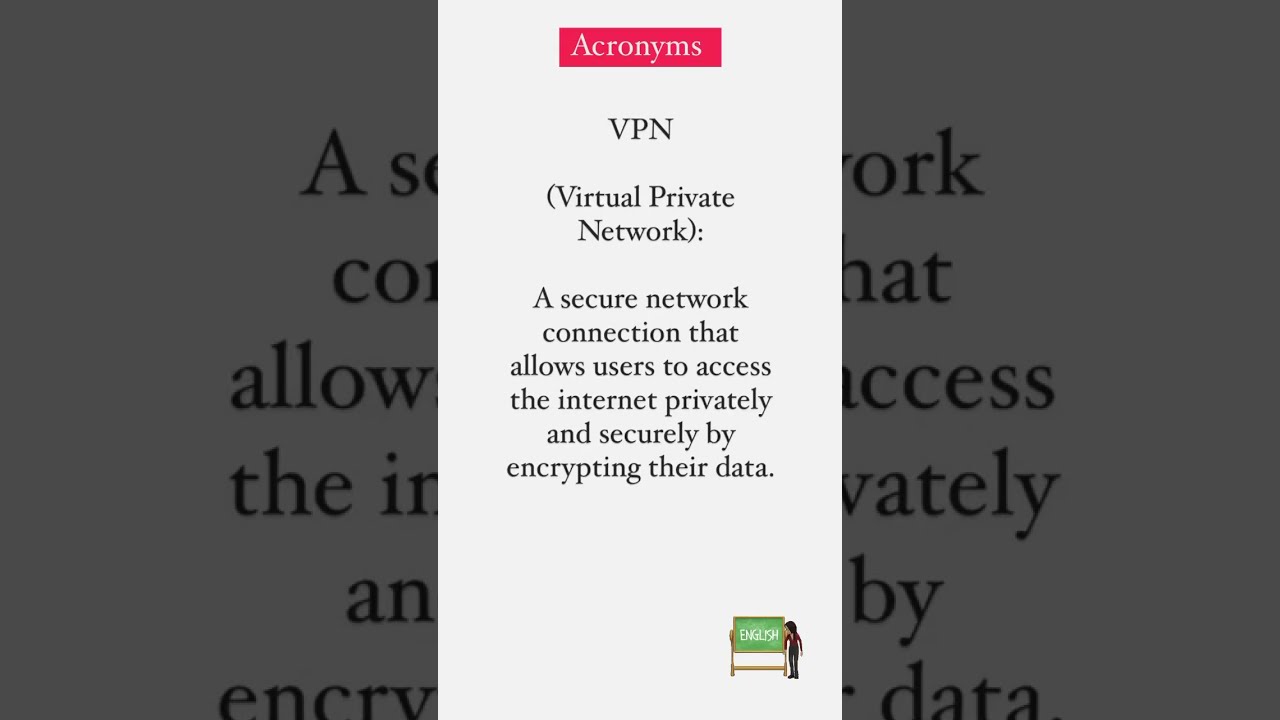The image appears to be a computer screenshot in a wide, horizontal rectangle format. The background consists of large, grayed-out text, where only a few scattered words like 'allow,' 'access,' 'privately,' 'encrypting,' and 'data' are legible, suggesting it repeats the same content as the central image. Dominating the center is a vertically oriented white rectangle featuring a detailed definition of 'VPN' in black text. At the very top of this central rectangle is a red box with white lettering that reads "Acronyms." Below, in black writing, it explains that VPN stands for Virtual Private Network, describing it as a secure network connection that allows users to access the internet privately and securely by encrypting their data. The bottom right of the central image displays the word "English." Additionally, there is a green chalkboard with a small figure standing next to it, visible in the background, complementing the overall instructional theme of the image.